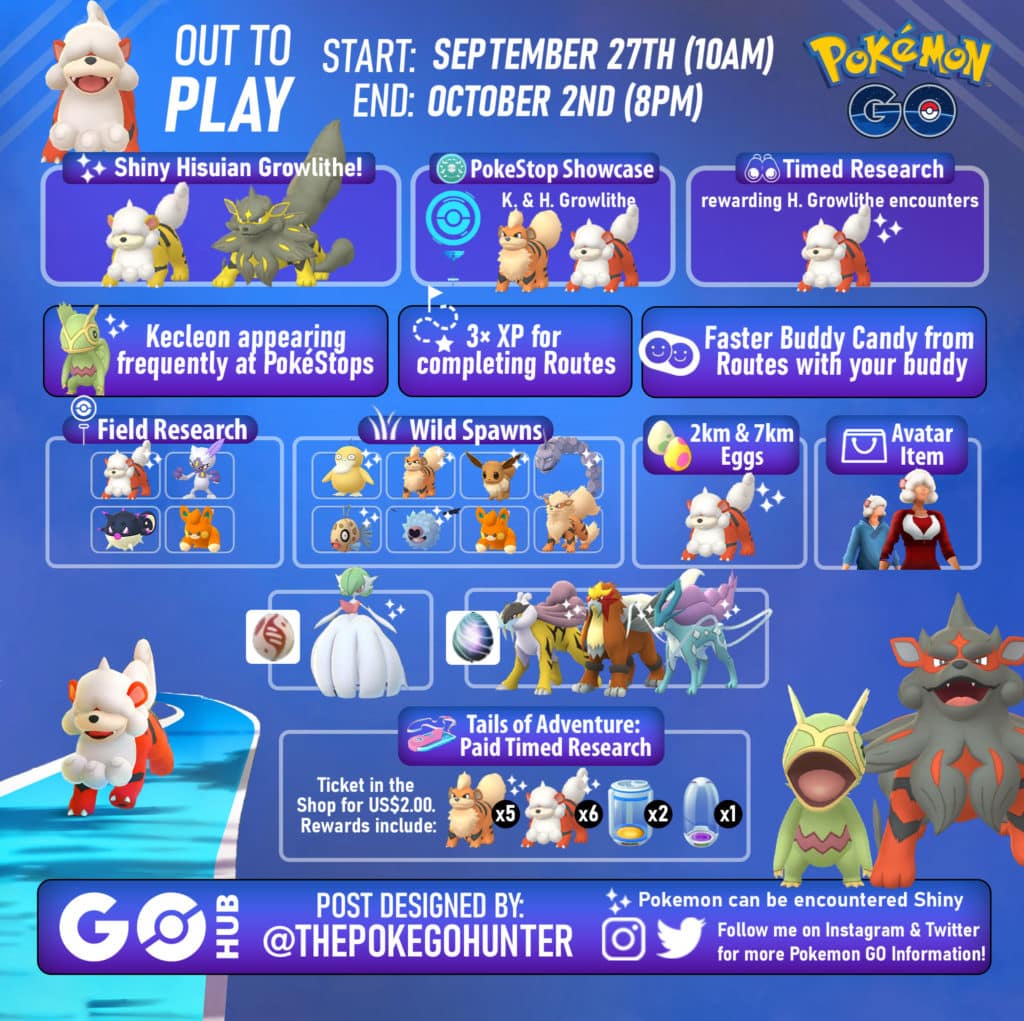**Event Poster for Pokémon GO: "Out to Play"**

The poster highlights the "Out to Play" event in Pokémon GO, scheduled to start on September 27th at 10 a.m. and ending on October 2nd at 8 p.m. The title "Out to Play" is prominently displayed, and the visual centerpiece features various Pokémon in the upper left corner, including an orange-and-white dog-like Pokémon, which resembles Hisuian Growlithe.

Key event details are broken down into various sections with rounded rectangular shapes and white text:

1. **Event Duration**:
   - Start: September 27th at 10 a.m.
   - End: October 2nd at 8 p.m.

2. **Hisuian Growlithe Spotlight**:
   - Shiny Hisuian Growlithe with two other Pokémon.
   - Timed research specifically targeting Hisuian Growlithe encounters.

3. **PokéStop Showcase**:
   - Kecleon, a green and yellow Pokémon with two legs and two arms, will appear frequently at PokéStops.

4. **Experience Points and Buddy Rewards**:
   - Triple XP for completing routes.
   - Faster buddy candy accumulation from routes with your buddy Pokémon.

5. **Field Research Tasks**:
   - Four different Pokémon featured for completing field research tasks.

6. **Wild Spawns**:
   - Eight possible Pokémon spawning in the wild, including:
     - Psyduck, a blue water-type Pokémon.
     - Onix, a gray rock-type Pokémon.
     - An orange Pokémon resembling a teddy bear.

7. **Egg Hatches**:
   - Special Pokémon available from 2K and 7K Eggs.

8. **Avatar Items**:
   - New items to customize player avatars.

9. **Exclusive Research**:
   - Ultimate or rare Pokémon encounters.
   - "Tales of Adventure" paid timed research available in the shop for USD 2.00, rewards include special Pokémon and items.

10. **Design Credits**:
    - Poster designed by PokeGoHunter and showcased on Go Hub.

Additionally, the poster mentions that Pokémon encountered during this event may appear in their Shiny forms, adding an extra layer of excitement for players.

This detailed poster provides comprehensive information on the diverse activities and rewards available during the "Out to Play" event in Pokémon GO, making it a can't-miss event for Trainers.